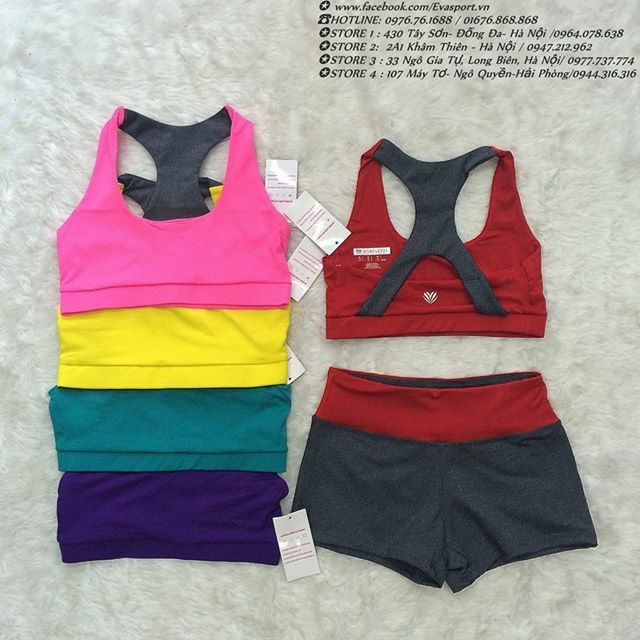This detailed photograph features an advertisement for women's sportswear set against a grayish white background reminiscent of a fuzzy carpet. At the top, the advertisement displays the website www.facebook.com/evasport.vn in black text. Below this, the image showcases a phone with the contact information "hotline: 0976.76.1688 / 01676.868.868". The advertisement lists four store locations numbered 1 through 4, each with specific details and phone numbers, though the text appears to be in an Asian language.

Prominently displayed in the image are multiple sports bras and one matching set of exercise shorts. On the left side, four colorful sports bras are aligned vertically. From top to bottom, the bras are hot pink, yellow, teal, and purple, each featuring a dark gray racerback design. To the right of these bras, there is a maroon/red sports bra paired with matching bottoms. The red sports bra is flipped to show the back, which crisscrosses in gray, matching the design element on the other bras. The accompanying shorts have a red waistband with gray bottoms. Each item has a white rectangular tag hanging from it. The sportswear is clearly organized to highlight the vibrant color options and distinctive design features.